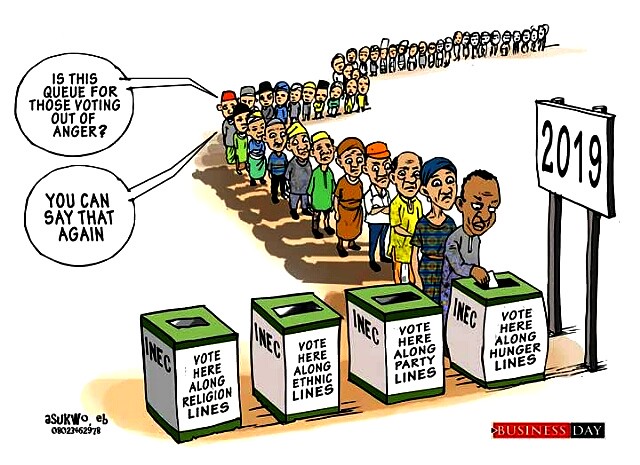This 2019 political cartoon, possibly by artist ASURKW0EB, depicts a long line of people waiting to vote, stretching off into the distance towards the upper right side of the image. At the forefront, the first person is seen placing a ballot into one of four boxes lined up on a table, which are labeled: "Vote here along hunger lines," "Vote here along party lines," "Vote here along ethnic lines," and "Vote here along religious lines." Notably, nearly all the people in line are queued up to cast their ballot into the "hunger lines" box. The ballot boxes bear the inscription "INEC" on the side. Two individuals in the line have a conversation, with one asking, "Is this queue for those voting out of anger?" to which the other replies, "You can say that again." The image carries a caption in the lower right corner, reading "A Business Day."